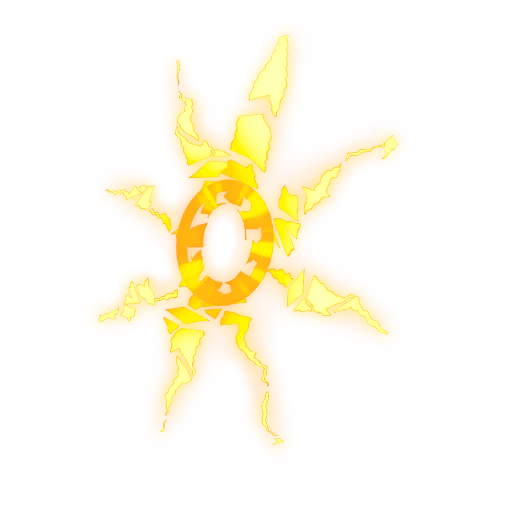This image features an artistic digital rendition of a sunburst set against a plain white background. At its center is a donut-shaped, dark orange ring with regular cutouts around its middle, subtly highlighted with lighter shades of yellow. Radiating from this ring are eight irregular, cracked rays resembling a sun's rays, rendered in a light yellow hue and finely bordered with orange that bleeds into the rays. These rays are broken into segments, creating a mosaic-like effect. The lengths of these segments vary, with three notably longer rays and the shortest ones positioned around the 8 and 9 o'clock positions. The entire composition gives a vibrant yet fragmented impression of a sunburst.